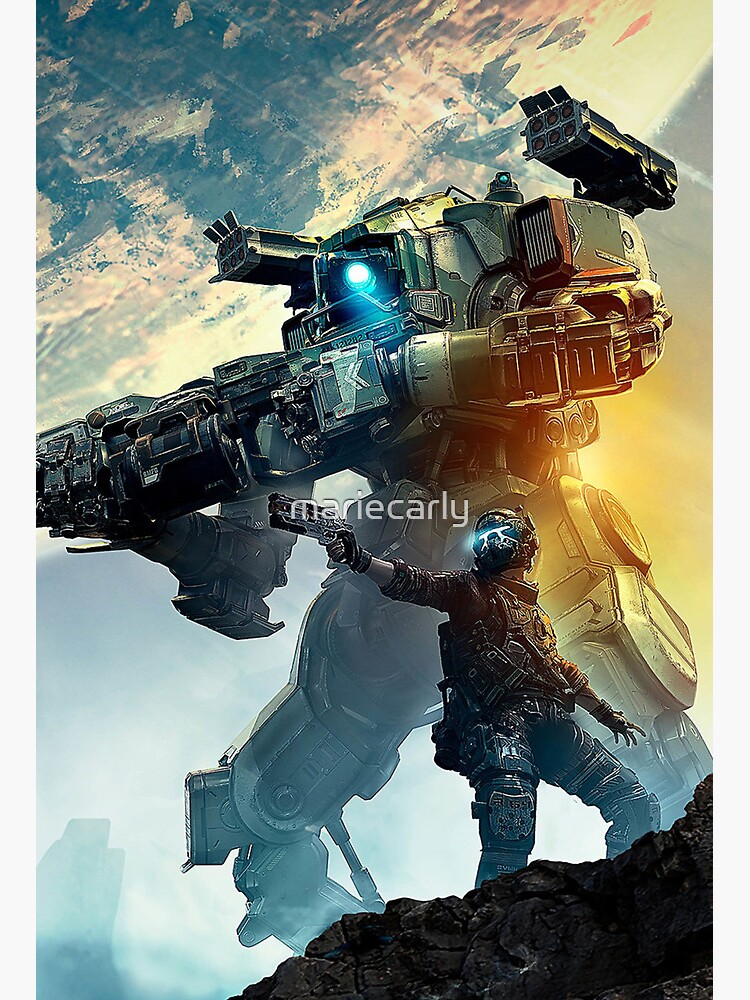The image appears to be a highly detailed, AI-enhanced or cartoonish movie poster or game artwork featuring a futuristic, action-packed scene. It depicts a man in full tactical gear standing on dark rocks, with his right arm extended and holding a handgun. He is wearing a helmet with a blue shining light in the face area, giving him a formidable, high-tech appearance. Positioned right behind him is a massive robot or mecha, towering at about three times his height. This robot is also equipped with artillery guns on its shoulders and holds a large machine gun, pointing it in the same direction as the man. The robot's face area also emits a blue light. The scene is set in outer space, with a large, blurry planet in white, tan, and charcoal gray hues looming in the background. Above the central figures, the name "Marie Carly" appears, hinting at either an individual artist's signature or a title. The characters and their gear, combined with the outer space setting and the large planet, give the artwork a strongly futuristic and action-oriented vibe, reminiscent of a movie or game advertisement.